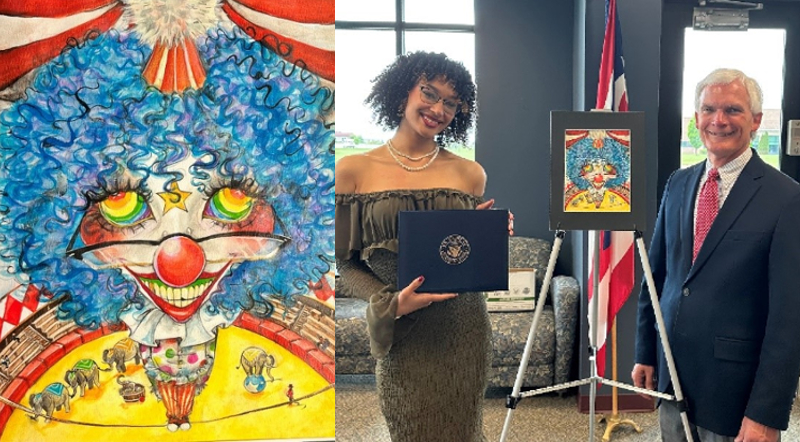The composite photograph consists of two images: on the left, a detailed close-up of a vibrant painting, and on the right, a scene of two individuals standing beside the artwork.

The left-hand side of the photo showcases a depiction of an exaggerated clown with prominent blue curly hair and a red hat adorned with a white pom-pom. The clown's face features rainbow-colored eyes, a large red round nose with a green star marked 'S', and a broad grin with yellow teeth and green gums. The clown is seen performing on a tightrope, wearing a polka dot shirt and red-striped pants. Below the tightrope, an intricate circus scene unfolds, complete with elephants performing tricks, a ringmaster, and an audience in the bleachers.

On the right-hand side, a white metal easel with a black mat holds the painting, set against a backdrop of a dark grayish-blue wall and a drooping flag suspended from a golden stand. The setting has a window on the left, a door on the right, and a gray floral-patterned couch beneath the window. A woman stands to the left of the easel, donning a low-cut brown dress, her medium-length curly brown hair framing her face with horn-rimmed glasses and a bright pink smile. She displays a blue diploma or award with both hands, her neck adorned with two lines of pearls. To the right and slightly behind the easel is a man in a blue jacket, white shirt, and red tie, grinning with short black hair. This scene conveys the celebration of winning an award for the clown painting, highlighting the joyful and proud moment of achievement.